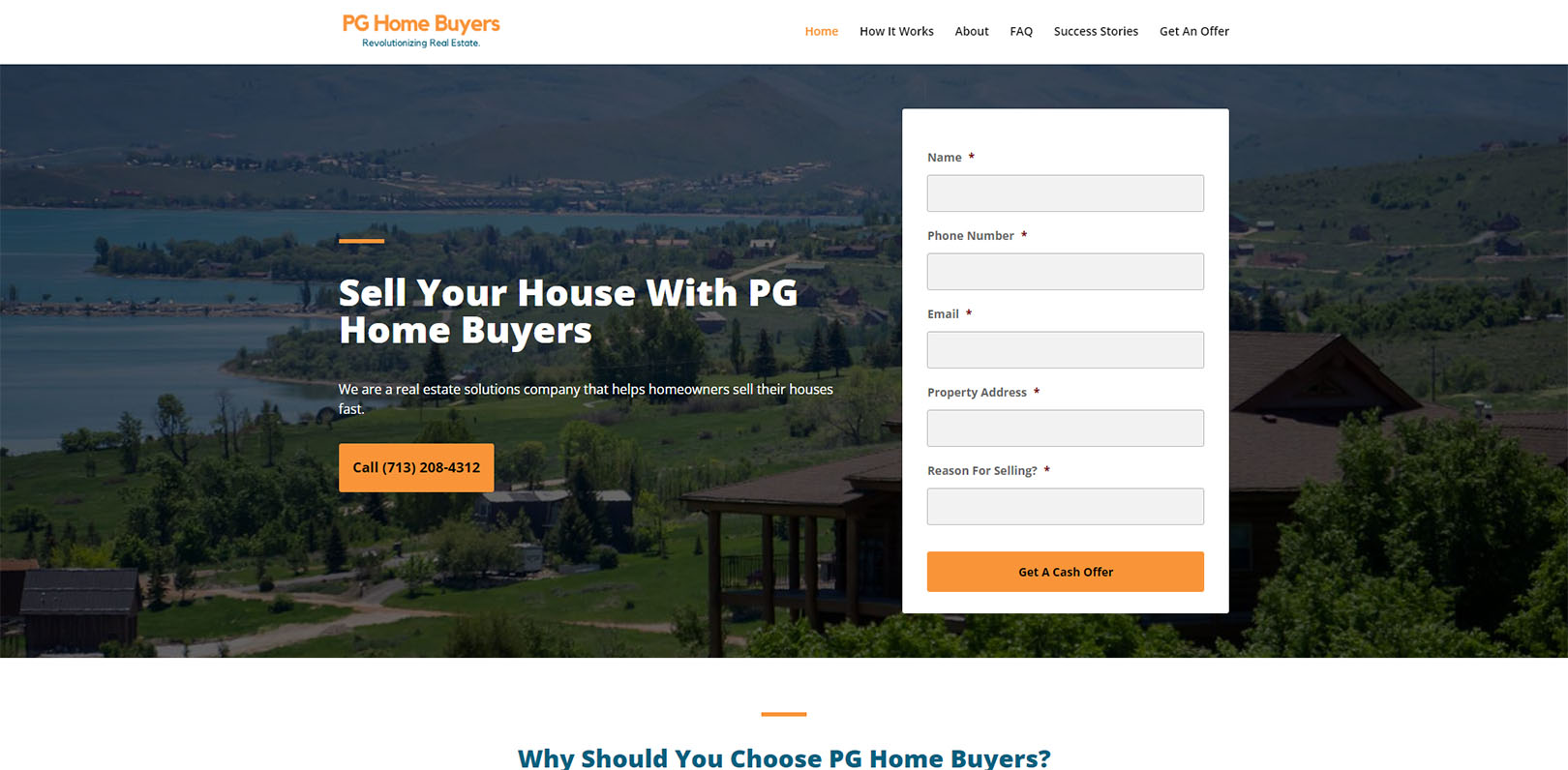The web page of PG Home Buyers, a revolutionary real estate solutions company, features a streamlined design to help homeowners sell their properties quickly. In the upper left corner, the company's logo and name are prominently displayed. 

A horizontal menu bar spans the top of the screen, listing menu options: Home, How It Works, About, FAQ, Success Stories, and Get an Offer. The "Home" option is highlighted in orange, indicating the current page.

The central part of the web page showcases a large, picturesque image of a lakeside town set against a mountain backdrop. The image is slightly darkened to accentuate the overlaid text. 

On the left side of the page, the heading "Sell Your House with PG Home Buyers" is prominent, followed by the subheading, "We are a real estate solutions company that helps homeowners sell their houses fast." Below this is an orange box displaying a contact number: "Call 713-208-4312."

Adjacent to this, there is an information box requesting user details including Name, Phone Number, Email, Property Address, and Reason for Selling. 

At the bottom of the form, a button labeled "Get a Cash Offer" invites users to submit their information.

Directly below the image, a caption reads, "Why should you choose PG Home Buyers," suggesting an introduction to the company's benefits and unique selling propositions.